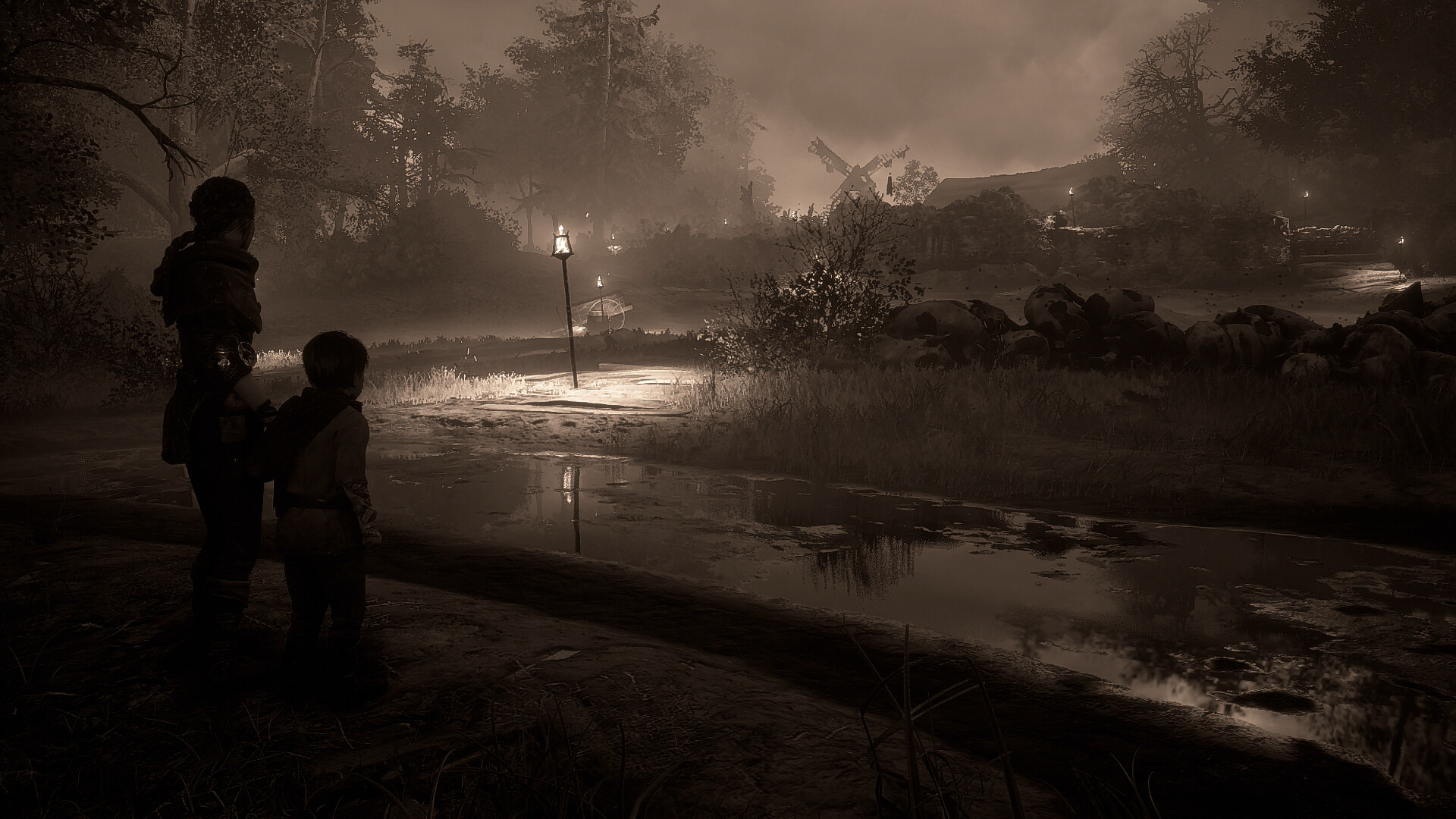The grayscale image, appearing to be a cinematic screenshot from a video game, captures a somber and overcast scene. In the foreground, a woman with long hair, likely configured in a ponytail, stands holding hands with a young boy with short hair. Both wear greyish-brown, ragged clothes, and their backs are toward the viewer as they gaze across a narrow, surface-water-laden path. The standing water glistens under a few illuminated street lights scattered around the scene. To their left, a light pole with a triangular-shaped light bulb sheds additional, gloomy light on the surroundings. The path leads past a patch of grass dotted with small bushes and rocks, eventually reaching a distant house nestled among numerous trees. Further details, like a windmill and a cottage further back, add depth to the woodland setting, suggesting a remote village beyond the immediate scene. The entire environment, characterized by mossy, dirty water and an overcast sky, hints at a recent rainstorm, amplifying the overall dreary mood.